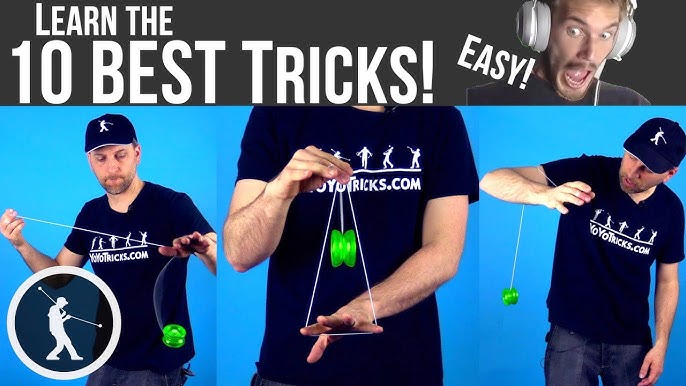The image is a thumbnail for a video, resembling a collage of photographs and text designed to catch the viewer's attention. At the very top, there is a dark gray, almost black horizontal border. On the left side of this border, white text reads "Learn the ten best tricks!" with "easy" written to its right. 

Below this border, a man wearing gray earphones is depicted looking downward, with an excited, open-mouthed expression. 

Beneath him, the main section of the thumbnail features three separate photographs of another man engaged in various yo-yo tricks. This man is wearing a black baseball cap and a black t-shirt that says "yo-yo tricks.com" in white text. The t-shirt also has silhouettes of men performing different yo-yo tricks.

In the first photo on the left, he is swinging a green yo-yo below his hands. In the middle photo, the yo-yo is forming a trapeze, swinging between its own string. In the right photo, the yo-yo is looped over his arm. 

At the bottom left of the image, there is a white circular logo featuring a stylized silhouette of a man facing right, swinging two yo-yos in opposite directions. The logo mirrors the logo on the man’s baseball cap and shirt.